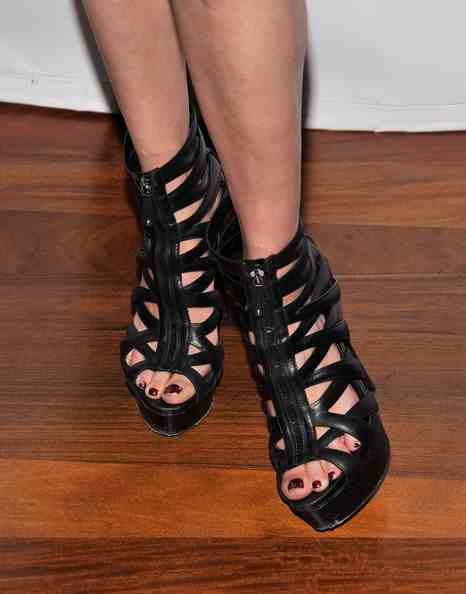The photograph is a close-up of a woman's feet, visible from just below the knees. She is wearing black, gladiator-style high heels with chunky platform soles. The heels feature multiple black leather straps that crisscross in an X pattern along the inner and outer sides of her feet, all converging at a zipper running from her toes to the front of her ankles. Her toenails, painted in a vibrant burgundy red, are peeking out from the open-toed sandals, with some of the polish noticeably chipping to reveal the natural pink nail underneath. The feet rest on a dark, red-stained wooden plank floor that occupies the bottom two-thirds of the image. In the top portion, a white fabric, likely from a bed or seating, creates a stark contrast against the dark floor.